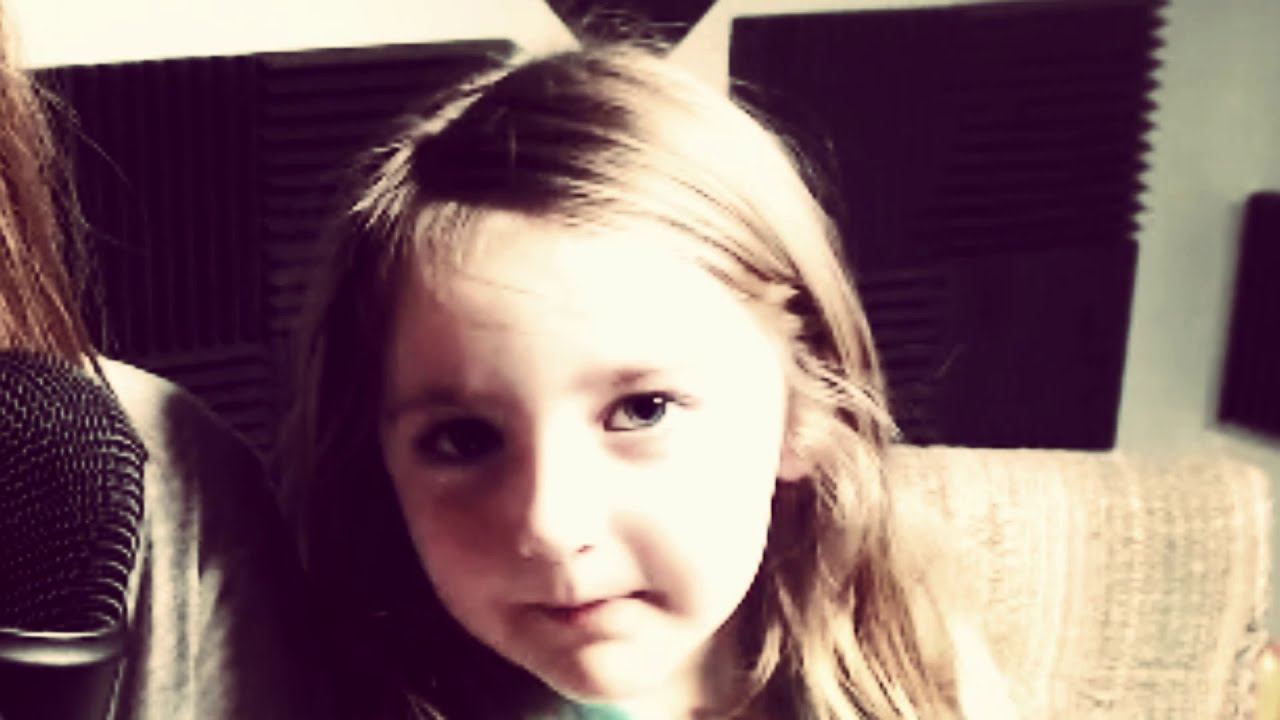This is a landscape-oriented, horizontal rectangular image that appears to be a colorized black and white photograph with a dark, low to poor quality, possibly sepia-toned filter. The central focus of the image is a young girl, about four or five years old, with long, blondish-brown hair styled with a side part and pulled back behind one ear. She is seated on a beige, brown, or tweed-like couch, looking directly at the photographer. Her face occupies most of the image, making it a close-up shot that highlights her eyes and facial features. The girl's green shirt adds a touch of color to the otherwise subdued palette of the scene.

Behind her, the background is dark, possibly featuring a television screen, framed photographs, or soundproofing material. There is also the presence of a boom microphone coming out from the lower left part of the image. To the left of the girl, there seems to be another person with shoulder-length light brown hair and a gray shirt, adding another element to the composition. Additionally, a pillow might be placed next to the girl on the couch. The image dimensions are approximately eight inches wide by five inches tall.